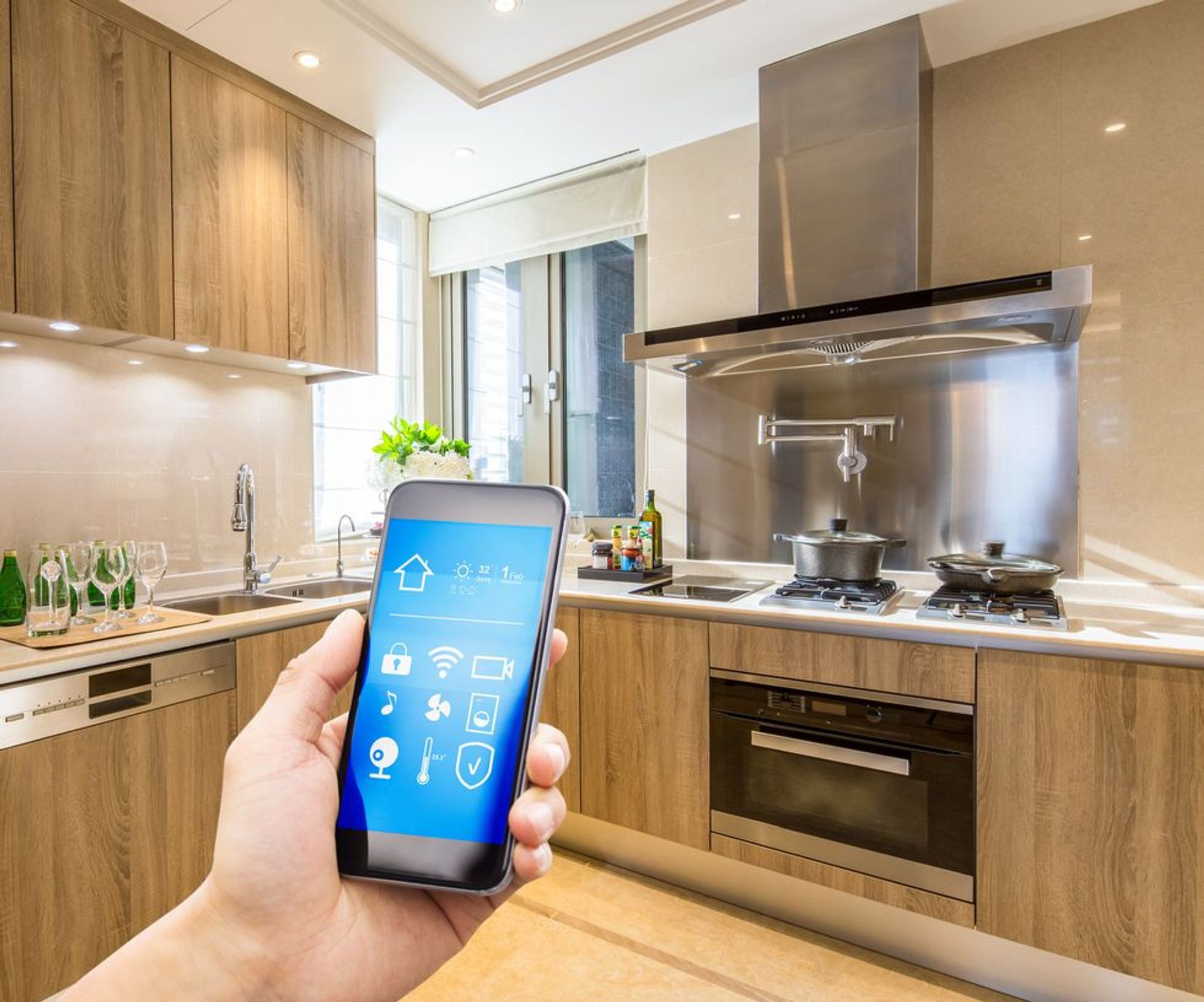This photograph captures a detailed view of a kitchen interior. In the lower left corner, a hand is partially visible, holding a black cell phone with its screen lit up. The phone display shows various icons, including settings, lock, and an arrow in the corner. The kitchen features medium-colored wood cabinetry, possibly oak, with upper and lower cabinets that have no visible hardware. On the right side of the back wall, there is a gas stove with four burners, crowned by a large, stainless steel exhaust fan that adds a modern, sleek touch to the space. In the left corner, a window fitted with white blinds is partially raised, allowing light to filter into the room.